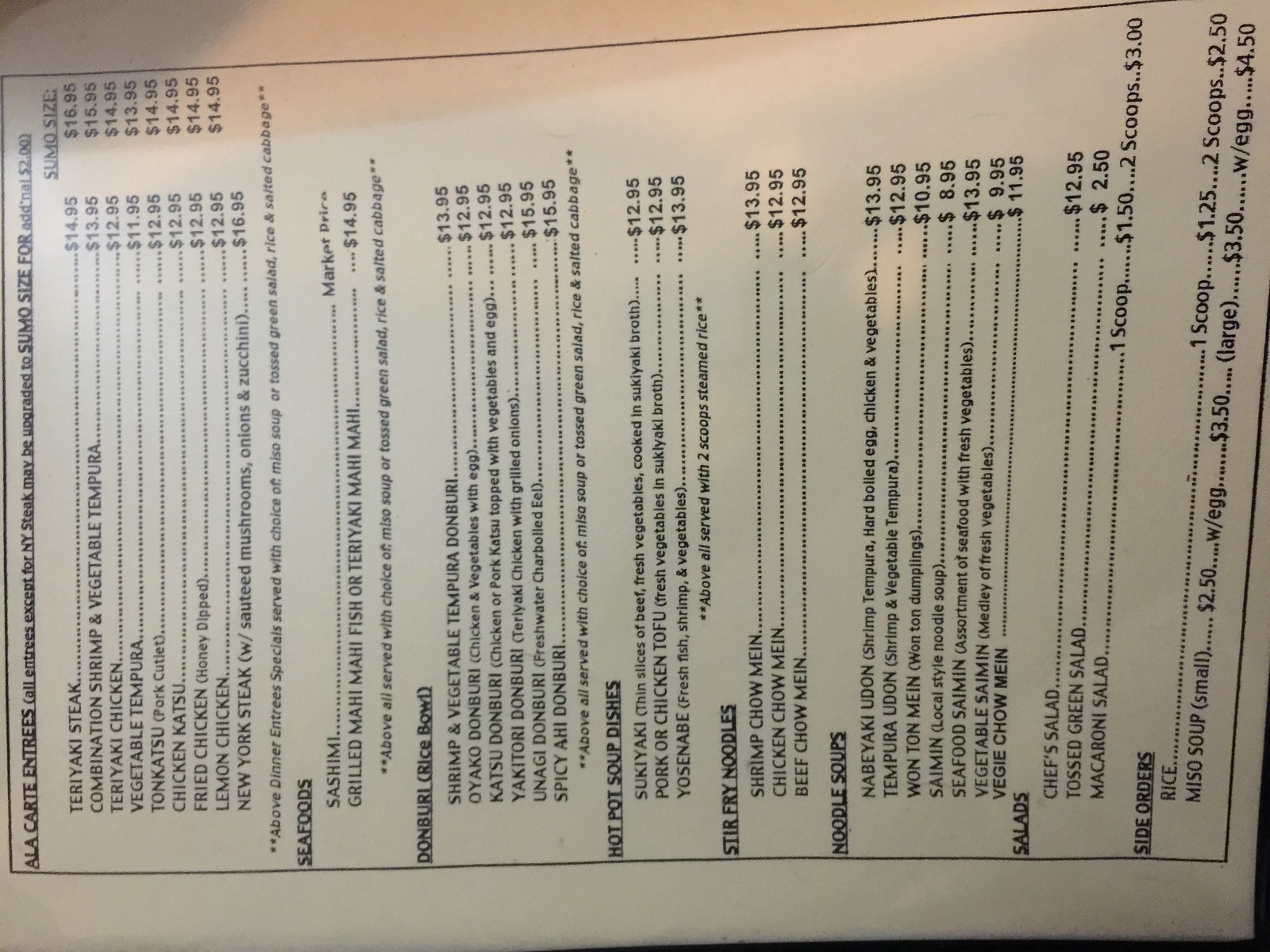This black and white image features a menu that appears to be oriented sideways, as if one were holding it and then rotated it 90 degrees to the left. To read the menu, one would need to tilt their head to the left. Displaying an array of a la carte entrees, the menu offers the option to upgrade most dishes (excluding New York State entrees) to "sumo size" for an additional $2. The categories featured include seafood, donburi (rice bowls), hot pot soups, stir-fried noodles, noodle soups, salads, and side orders such as rice and miso soup. 

Highlighted items under a la carte entrees are teriyaki steak, a combination of shrimp and vegetable tempura, and teriyaki chicken. Notable seafood options listed are sashimi, grilled mahi-mahi, and teriyaki mahi-mahi. The rice bowl (donburi) section includes dishes like shrimp and vegetable tempura donburi priced at $13.95, and yakitori donburi, which consists of teriyaki chicken with grilled onions, priced at $12.95.